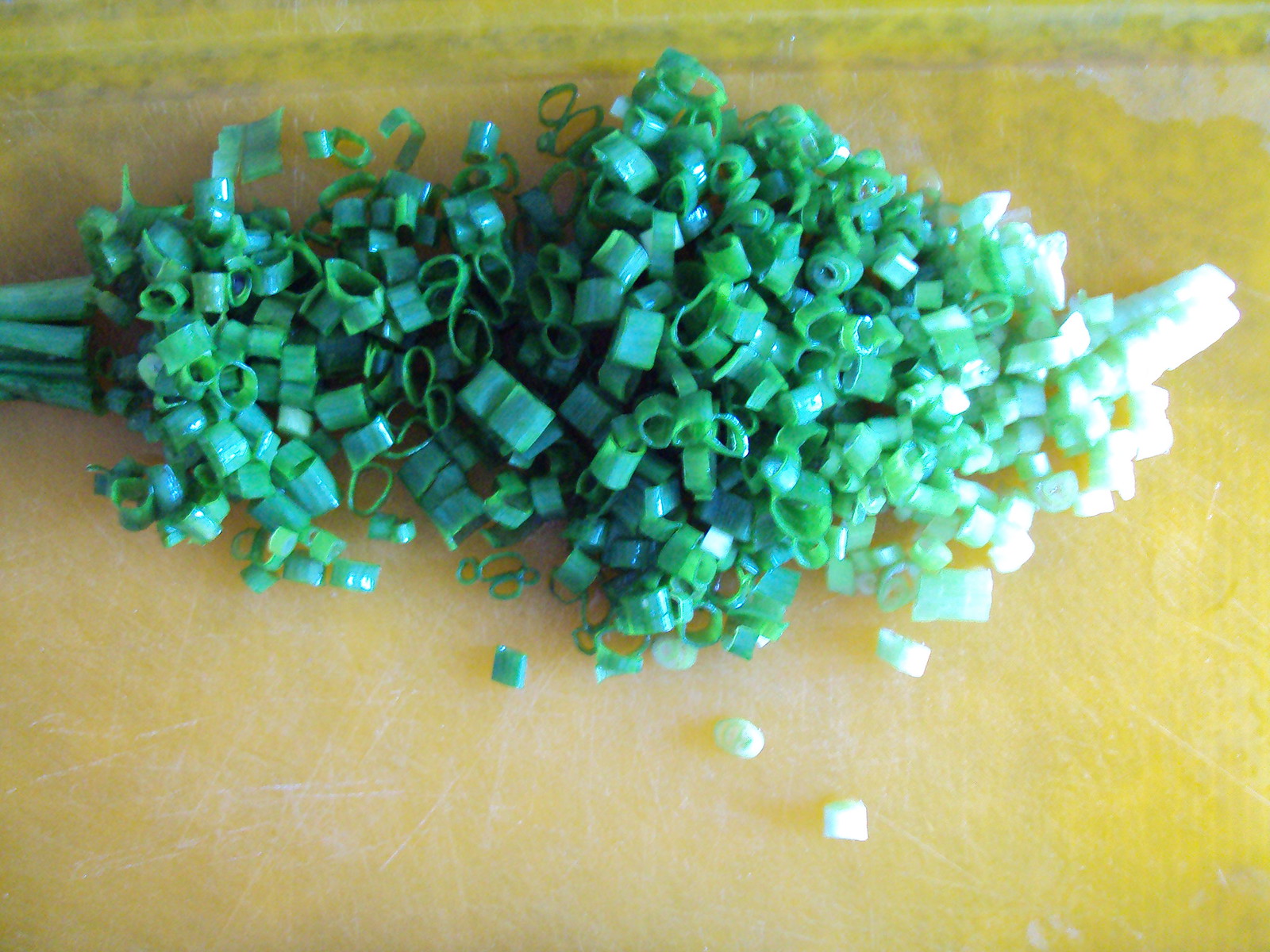This image provides a detailed, downward view of a well-used, light yellow chopping board adorned with numerous scratches and slight staining along the top edge. On the cutting board lies a large pile of freshly chopped green onions, creating a gradient from the vibrant green tops on the left to the white bulbs on the right. The uncut ends of the green onions are also visible on the left-hand side. The chopped onions maintain their characteristic circular shape, forming tubular rings. Some stray pieces have fallen loosely around the main pile. Bright light from the right side overexposes the white parts of the onions, making the details hard to discern. The board's surface features a border along the top and bottom edges.